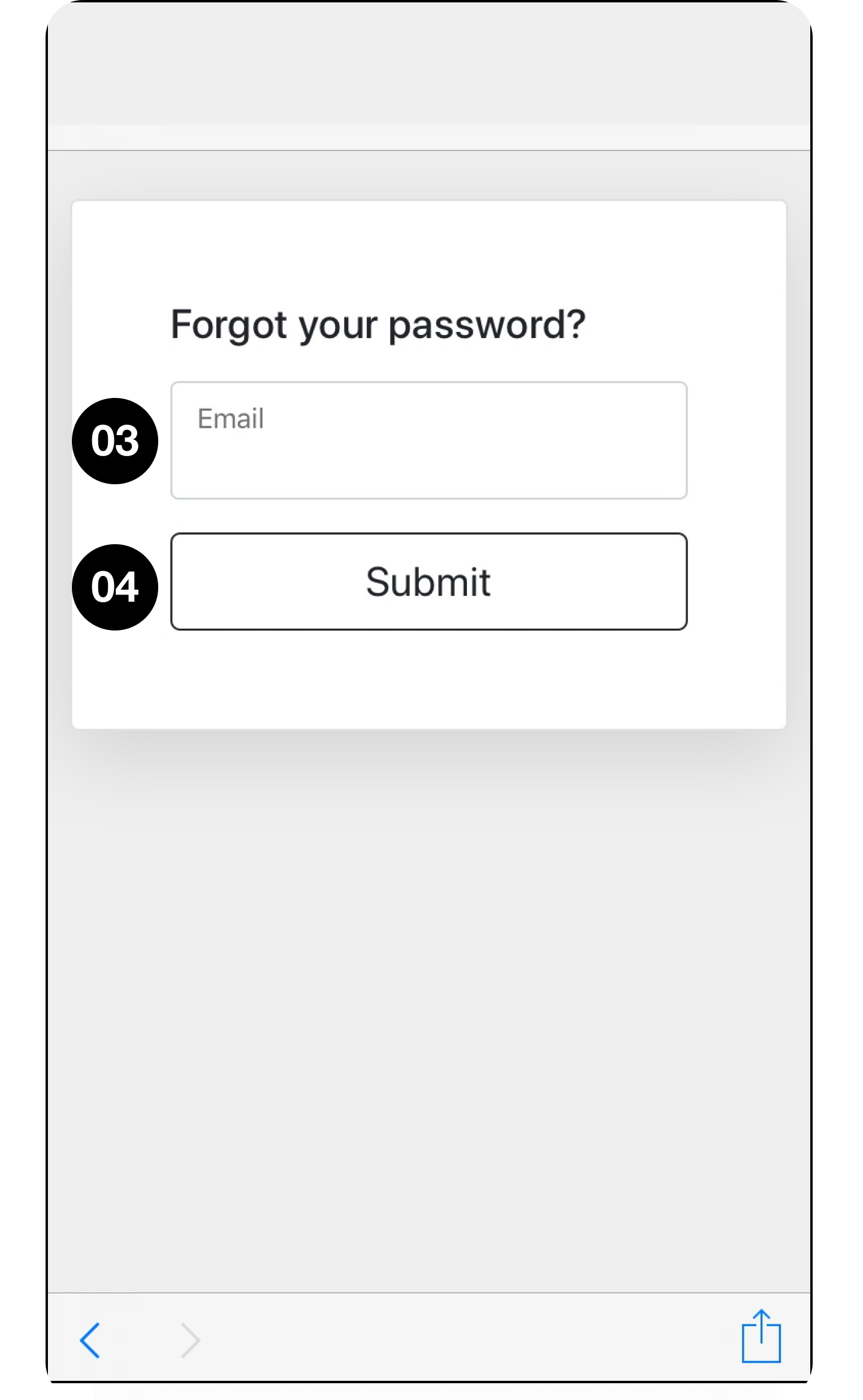Screenshot of a mobile phone screen, meticulously outlined by a thin black border against a gray background. The screen features a minimalist design, starting with a top bar in plain gray, delineated by thin horizontal lines above and below it. The bottom of the screen is bordered by a similarly thin line above a light gray bar. This bar contains navigation icons: a blue left-facing arrow on the left and a gray right-facing arrow on the right. Located in the lower-right corner is a distinctive blue square 'send' icon with an upward-pointing arrow emerging from its center.

Dominating the upper portion of the main screen area is a large white rectangle displaying black text that reads "Forgot Your Password." Below this prompt, there are two interactive elements: first, a text entry box for the user's email, marked by a black circle containing the number '3,' and second, a submit button, identified by a black circle with the number '4' within it.